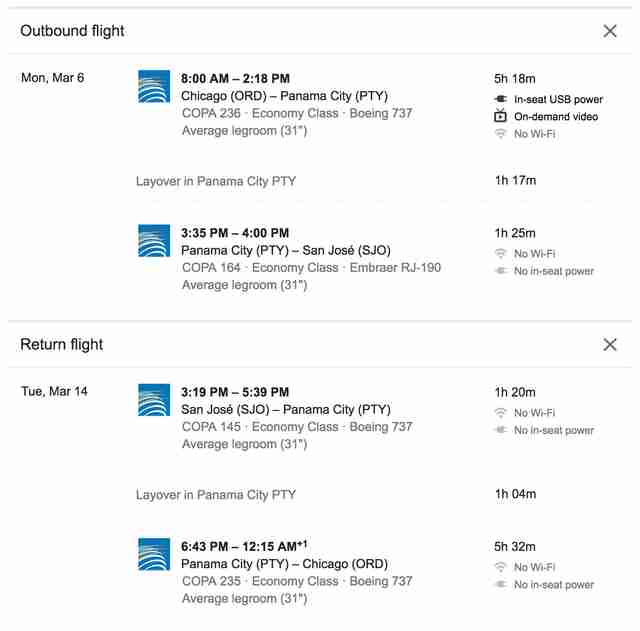This screenshot depicts the flight itinerary for a trip, showcasing the details of outbound flights. At the top left, the title "Outbound Flights" is displayed, and there is an 'X' icon on the far right for closing the screen. Below the title, the date "Monday, March 6" is indicated on the left. The itinerary lists two flights, each accompanied by a small thumbnail of the airline's logo.

The first flight details are as follows: 
- Departure at 8:00 AM and arrival at 2:18 PM
- Route: Chicago to Panama City
- Airline: Copa Airlines, Flight 236
- Class: Economy
- Aircraft: Boeing 737
- Additional information: Average legroom of 31 inches

On the right side, the flight duration and amenities are noted:
- Flight duration: 5 hours 18 minutes
- In-seat USB power
- On-demand video available
- No Wi-Fi service

Following this, there is a layover in Panama City.

The second flight details include: 
- Departure at 3:35 PM and arrival at 4:00 PM
- Route: Panama City to San Jose
- Airline: Copa Airlines, Flight 164
- Class: Economy
- Aircraft: Embraer RJ 190